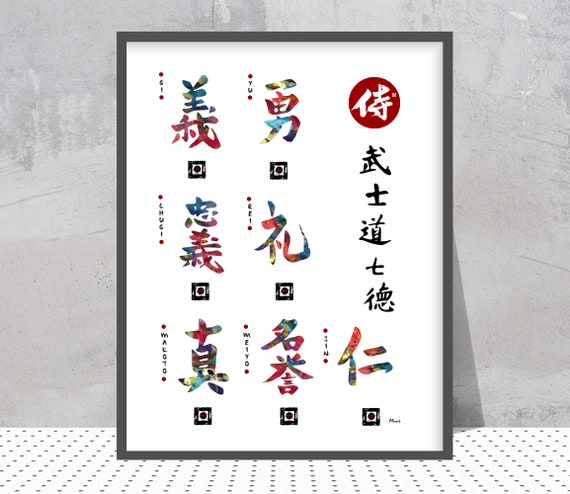This vertically rectangular poster features multi-colored, primarily rainbow-colored Japanese text within a black frame against a white background. Inside the frame, the text is arranged in two vertical columns and several horizontal rows, with words like "GU," "SHUGI," "REI," "MAYOTO," "MIYO," and "JIN." Pronunciations for some characters appear as "Ray" and "Mayo." The poster is propped up against a gray wall, casting a shadow on the wall’s lower right part. It rests on a white surface adorned with vertical blue dots. Additionally, there is a white metal grate at the bottom of the image and a red circle followed by five script letters along the right side of the poster. There are no people, watermarks, or additional text present in the image.